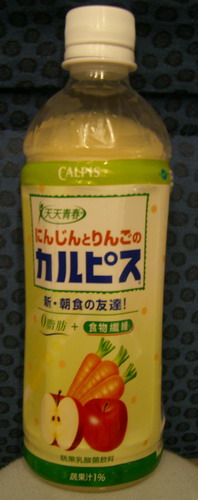The photograph features a tall, thin, transparent plastic bottle with a white screw-on cap, placed on a white surface against a dark gray backdrop with black dots. The bottle contains an off-white liquid, possibly a type of fruit and vegetable juice. The label on the bottle showcases a green trim at the top, with the English text "Calpis," likely referring to the company or product. The main label underneath is predominantly white with sections of foreign writing that resemble shapes or an Asian language, interspersed with some blue letters. At the bottom part of the label, there is a detailed illustration comprising a whole red apple, a sliced red apple displaying two seeds and a stem, three orange carrots with green tops, and what appears to be a tomato.